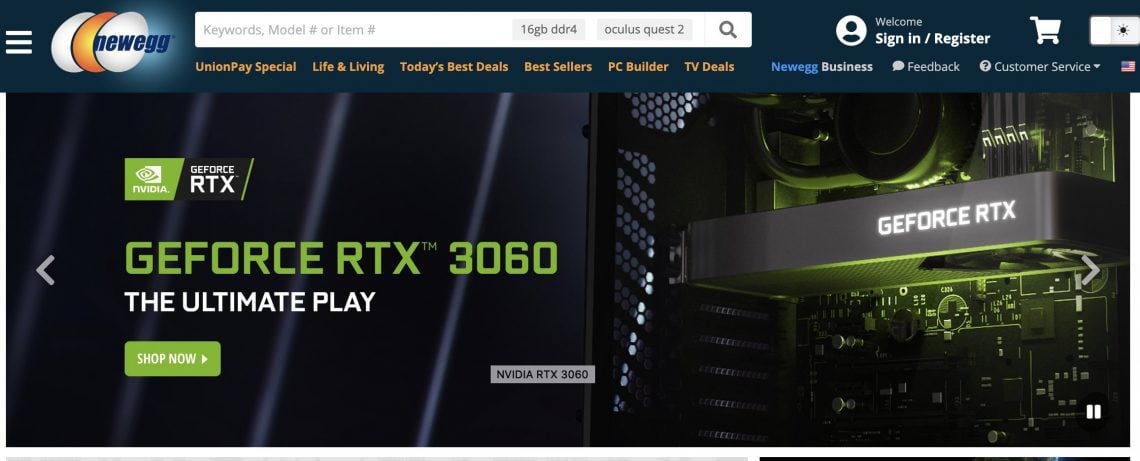This is a detailed depiction of the Newegg website's homepage layout. The Newegg emblem is prominently featured, consisting of a sequence of three eggs—white, orange, and white. The final white egg contains the word "newegg" in lowercase and navy print. 

At the top of the website, you'll find a search bar prompting users with options such as "keywords," "model number," or "item number." To its right, text examples like "16GB DDR4" and "Oculus Quest 2" appear, accompanied by a gray magnifying glass icon for initiating searches.

Continuing to the right, you are welcomed with a greeting text "welcome" and options for users to "sign in/register." A white, empty shopping cart icon is also visible in this section.

As you scroll down, a featured product section comes into view, showcasing the "GeForce RTX 3060" graphics card with the tagline "The Ultimate Play." Directly beneath, a green box with a white "Shop Now" text and an arrow pointing to the right encourages users to make a purchase.